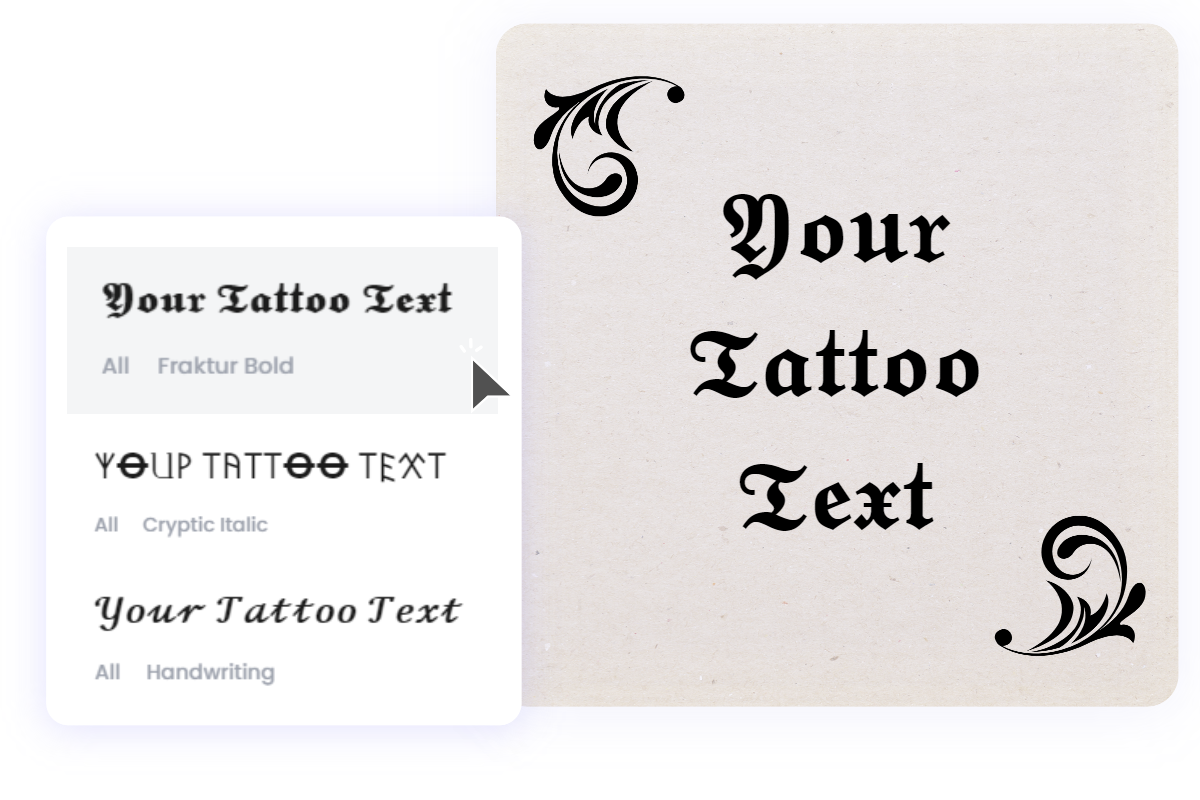The image features a comparative display of tattoo font examples on an off-white, creamy background. Central to the image are two squares aligned next to each other, with the larger gray square on the right and the smaller white square on the left. The gray square, decorated with intricate, fern-like flourishes curling downward, showcases the phrase "your tattoo text" in a sophisticated, old-English style font. In each of its corners, a curled fern design mirrors each other, adding to the ornate look. 

The white square on the left resembles a text input box with a blinking cursor at the top, inviting users to enter "your tattoo text" as if on a computer screen. Below the input area, several font options are listed: Fractur Bold, Cryptic Italic, and Handwriting, all presented in their respective styles. The Fractur Bold font mirrors the main example text on the gray square to its right, while Cryptic Italic appears like a series of almost Aztec-like symbols, and Handwriting is shown in a cursive script. The layout suggests a tattoo design tool, offering various font choices displayed as they would appear in a tattoo.